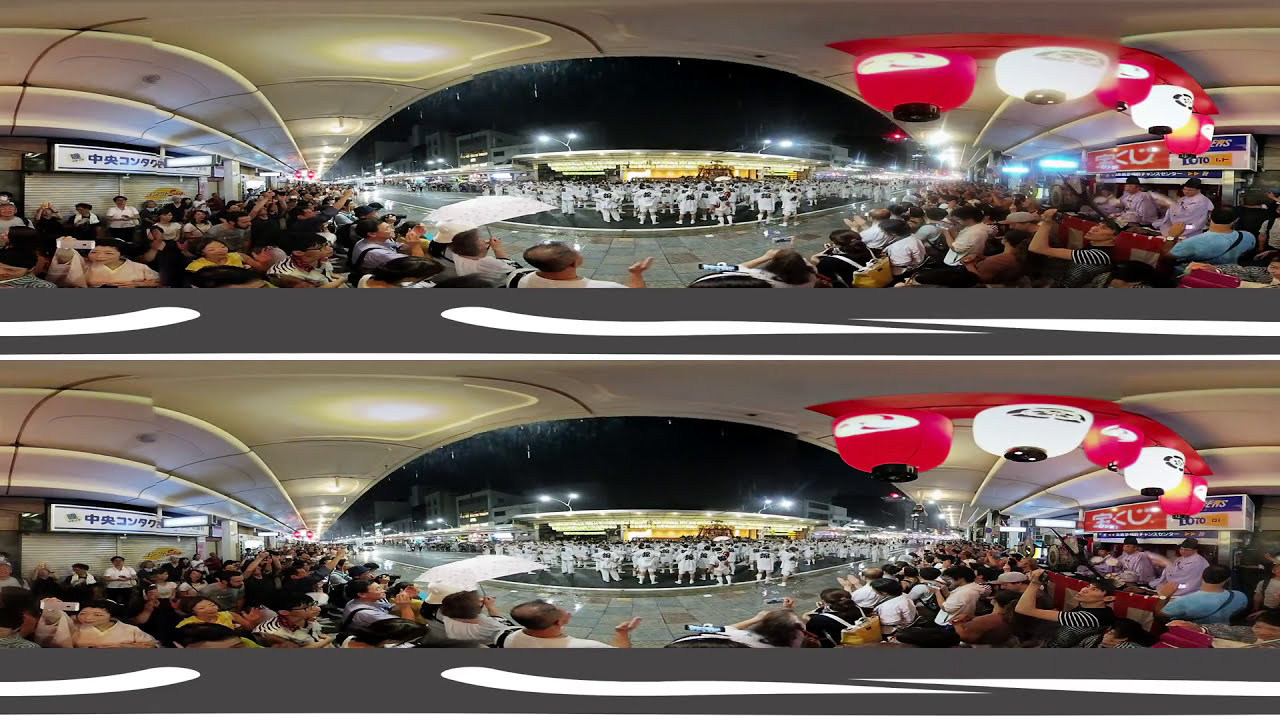The image features two nearly identical panoramic photographs stacked vertically, each composed of three perspectives from the same night-time event. Both photographs depict the view from inside a building, looking out toward a bustling street scene dominated by rows of people dressed in white uniforms, possibly part of a performance or a marching band. This contingent is standing on a well-lit road, set against the backdrop of another illuminated building and a pitch-black sky.

In the foreground, within the building, numerous spectators are visible, mainly their backs turned to the camera, as they focus on the outdoor event. Many are clapping, indicative of their engagement with the performance. Lanterns, six in total, hang on the right side of the image, featuring an Asian Oriental aesthetic with red and white hues.

The photographs also capture some unique details: a sign with black foreign text on a white background visible on the wall, and red-and-white lanterns resembling upside-down illuminated umbrellas. The composition intertwines elements like a dark green courtyard and intricate lighting, further emphasizing the vivid realism and representational style of the panoramic photography.